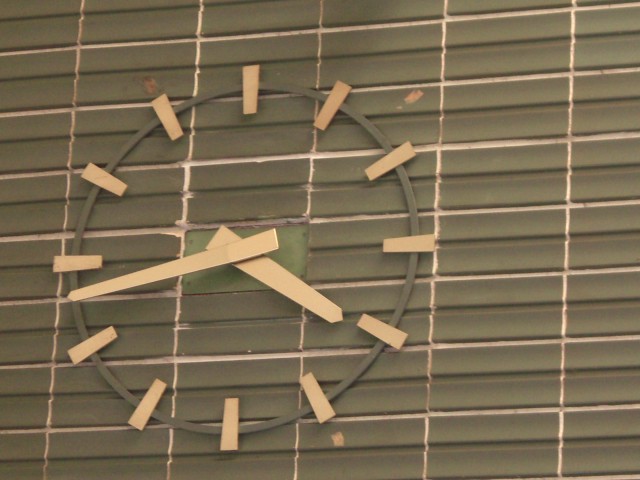This image depicts a large clock mounted on a wall. The wall is structured with various segments, including plastic blinds in a dark green shade, and has tan horizontal and vertical dividing lines, giving it a segmented, rectangular appearance. The clock itself is a significant circular structure, potentially covering an area as tall as nearly five stories. Unlike typical clocks, it features no traditional numbers; instead, tan lines or triangular pieces of wood represent the hours. The clock's hands are also tan in color, and the current time displayed is approximately 4:43. The wall's design and the clock's minimalist approach to indicating time contribute to an intriguing and somewhat ambiguous visual presentation.